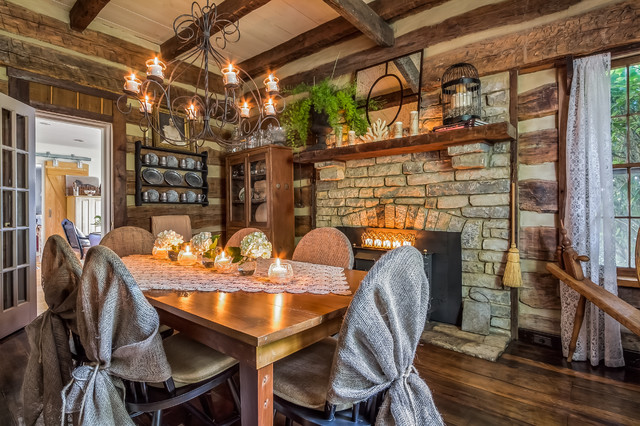The image depicts a richly appointed dining room in an older house, predominantly constructed of wood and stone. The shiny wooden floor and the wooden beams that support the ceiling add to the rustic charm. At the center of the room is a robust wooden dining table, draped partially with a white tablecloth. Arranged around this table are six chairs, each adorned with gray seat back coverings made of a straw-like material. Atop the table, three to four candles provide a warm, inviting glow, with additional illumination from a chandelier hanging gracefully above, featuring lit candles. 

Dominating the background is a stone fireplace with a metal insert for the wood fire, adding a cozy touch to the room. To the right of the fireplace, a broom stands ready for use, and a window with white blind drapes or curtains pulled back casts natural light into the space. The walls are made of wooden planks, and wooden frames border the windows and white door on the left side of the room. A small cabinet is tucked into the corner, adding to the room’s functional and aesthetic appeal.